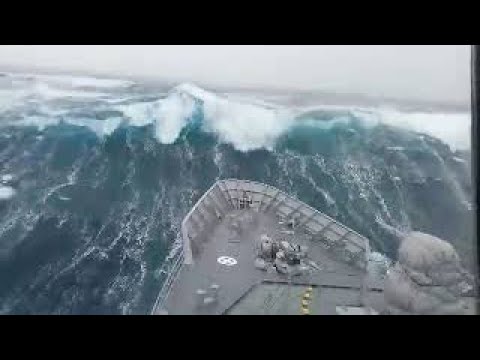The photograph depicts a large, gray battleship confronting an immense, dark turquoise and gray wave, capped with white foam, which appears taller than the ship's deck. The scene is stormy, with the turbulent sea evident in the white-capped waves stretching into the background. The image, seemingly captured from a high vantage point such as a mast or possibly a low-resolution security camera, has a dated quality, reminiscent of footage from a video game or an action movie due to its pixelation and lack of sharpness. The ship, featuring a prominent black and yellow stripe in the center and possibly carrying cargo, is shown at the bow. Black bands frame the top and bottom of the photograph, with a lighter area at the top that might suggest a distant shoreline, further emphasizing the perilous, rough waters.